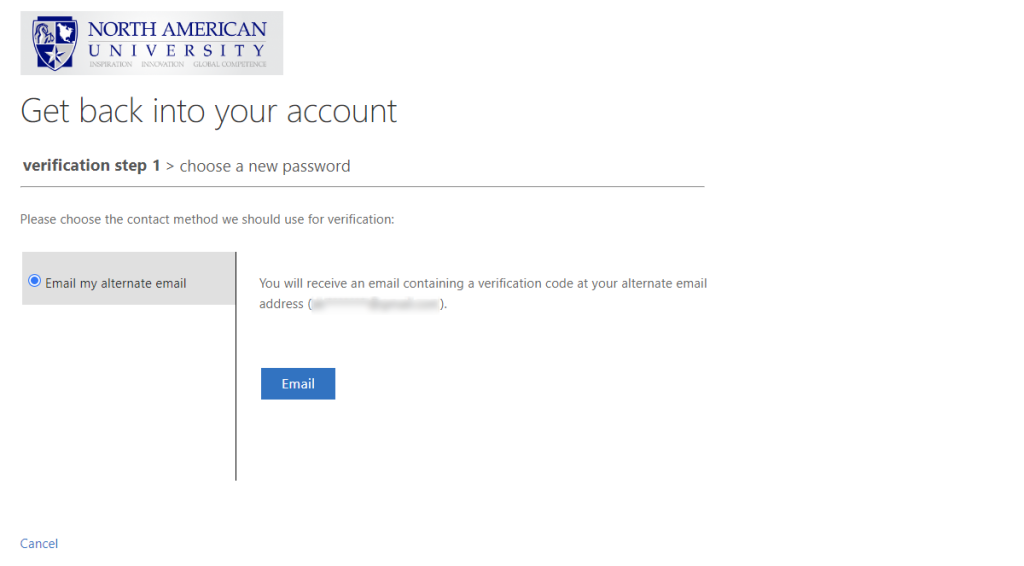Caption:
"A screenshot of the North American University account recovery page. The screen prompts the user to choose a new password as part of the verification process. The user is instructed to select a contact method for verification, with 'Email my alternate email' being the chosen option. A note indicates that a verification code will be sent to an alternate email address, which is partially blurred for security. Below the instructions, there are two clickable buttons labeled 'Email' and 'Cancel.'"